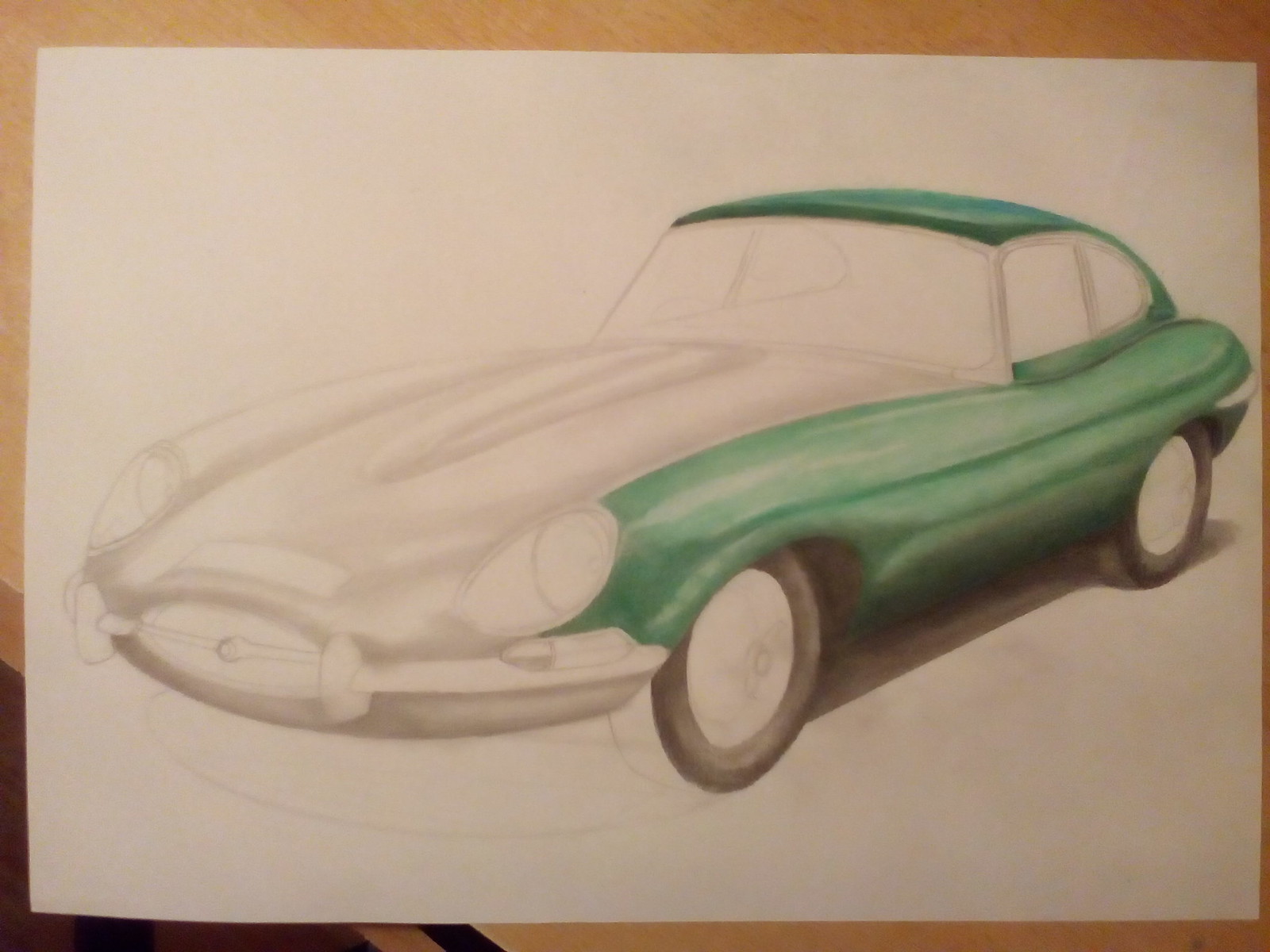This photograph features a close-up of a hand-drawn sketch of an old-fashioned car, most likely resembling a 1950s to 1970s Corvette or a similar sports car from that era. The drawing appears to be done in pencil on a white sheet of paper, which is placed on a light-colored wooden tabletop. The car is depicted in a semi-colored state; the right-hand side of the car, including part of the fender and the roof at the back, is painted in a seafoam green or silver color. The rest of the car, particularly the long front hood, headlights, bumper, and windshield, remains uncolored and only shaded in pencil. The black tires are the most detailed part, fully shaded in for emphasis. The photograph is amateur yet decently framed, with the image showing a dark brown table leg against a similar colored floor in the bottom left corner. There are no signatures or text indicating the artist, giving it an unfinished yet nostalgic look.